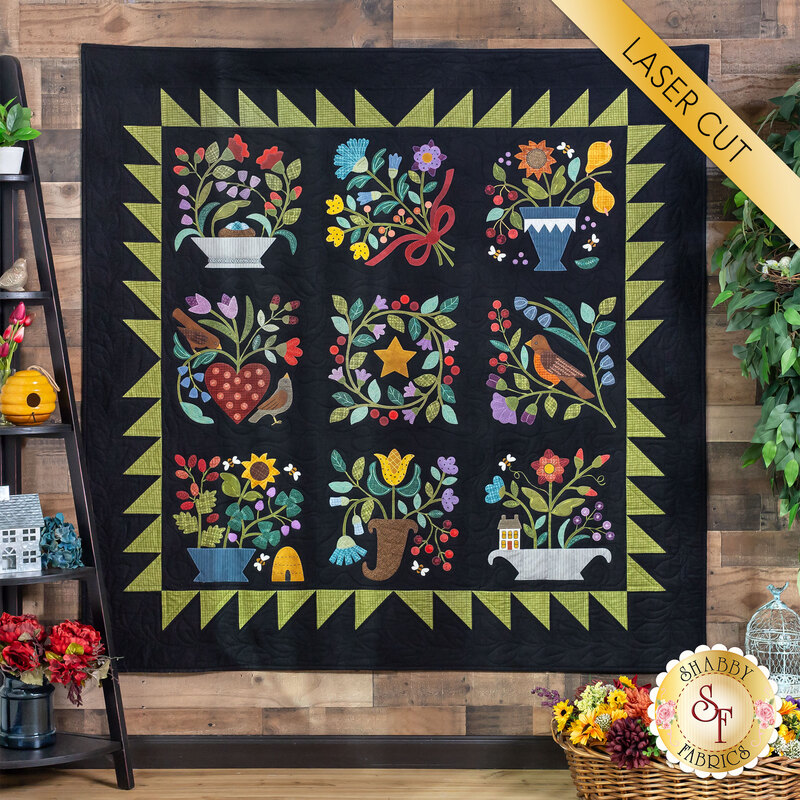This indoor photograph captures a detailed scene dominated by a large quilt displayed on a wooden wall. The wall itself is made of brown wood, seamlessly blending with the wooden floor. The quilt, which appears to be an advertisement for Shabby Fabrics SF, has a striking black background adorned with a border of green triangles that resemble sharp points or sunrays. Within this border, the quilt features an intricate array of embroidered designs showcasing a variety of floral and bird motifs. In the top-left square, there are red flowers, adjacent to a bouquet of blue, purple, and yellow flowers. Another section features a blue pot with orange plants and yellow pears, and nearby, a bird is perched on branches with red berries. Other designs include potted plants, a cornucopia of flowers, bees, a ribbon-tied bouquet, and a star encircled by a wreath of flowers and berries.

To the left of the frame, a ladder-like shelf displays various decorative items, while on the right, a basket brimming with flowers rests on the floor. In the top-right corner of the image, a yellow strip positioned diagonally reads "laser cut," and at the bottom-right corner, a circular logo states "Shabby Fabrics SF."